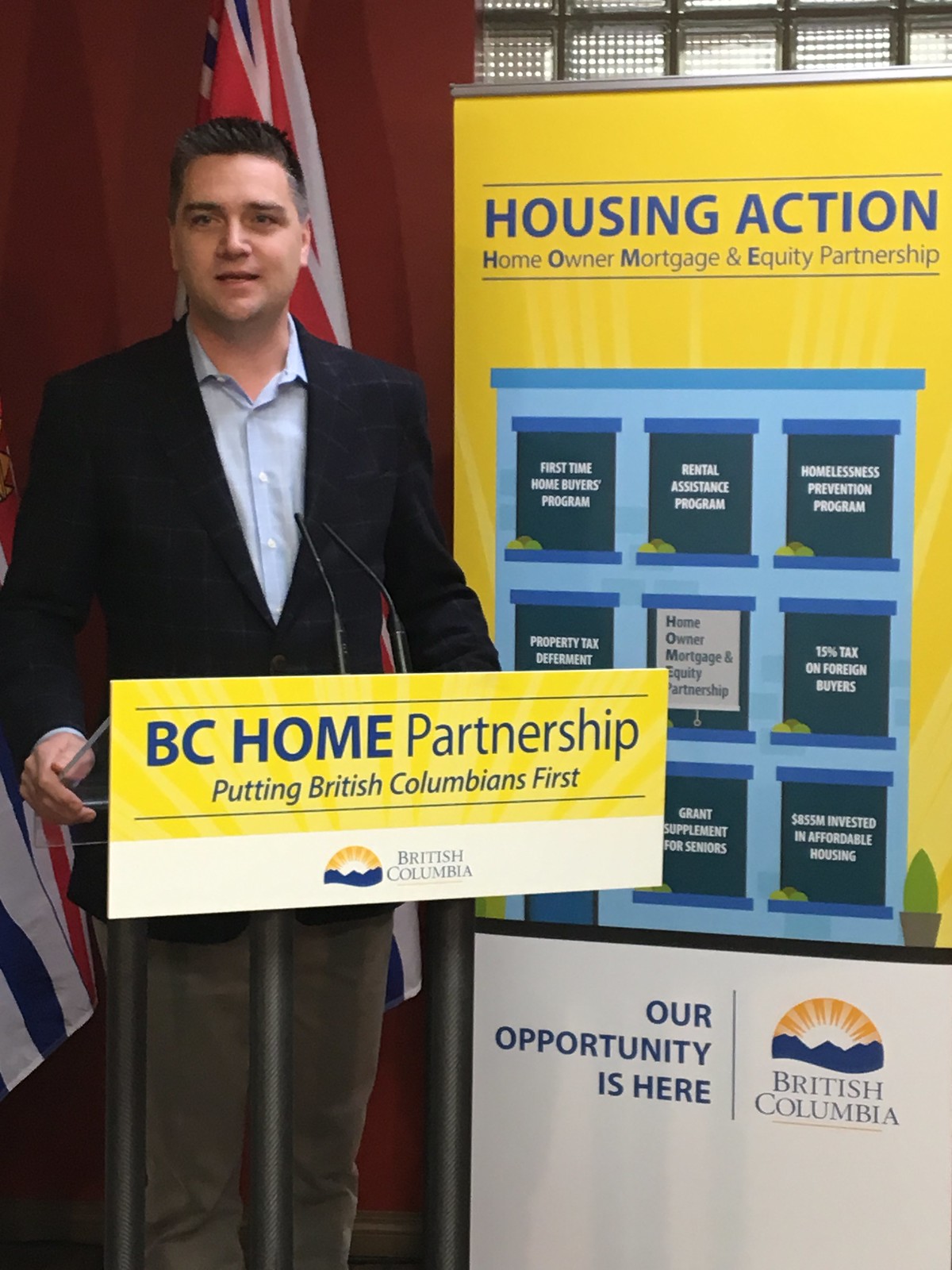This detailed color indoor photograph captures a white male with fair skin and short dark hair with gray on the sides, standing at a glass podium supported by metal pillars, equipped with two slim microphones. He is dressed in a black blazer over a light blue, unbuttoned collared shirt, without a tie. His brown pants contrast subtly with his attire. The podium features a yellow and white horizontal rectangular sign with blue lettering, reading "BC Home Partnership, putting British Columbians first," accompanied by a rising sun icon symbolizing British Columbia.

To the man's right stands a tall yellow sign titled "Housing Action, Homeowner Mortgage and Equity Partnership," adorned with a blue house graphic containing white-window texts. It lists various programs and initiatives including: "First-time Homebuyers Program, Rental Assistance Program, Homelessness Prevention Program, Property Tax Deferment, 15% Tax on Foreign Buyers, $855 million invested in affordable housing, Grant Supplements for Seniors." The sign is topped with "Our Opportunity is Here" in white text, accompanied by the British Columbia rising sun icon and name.

A flag featuring white, blue, and red colors hangs behind the man, set against a background that includes a brown wall and glass tiles on the right. This setting suggests an official or formal event related to housing initiatives in British Columbia, reflected in the extensive information displayed both on the podium and the adjacent sign.